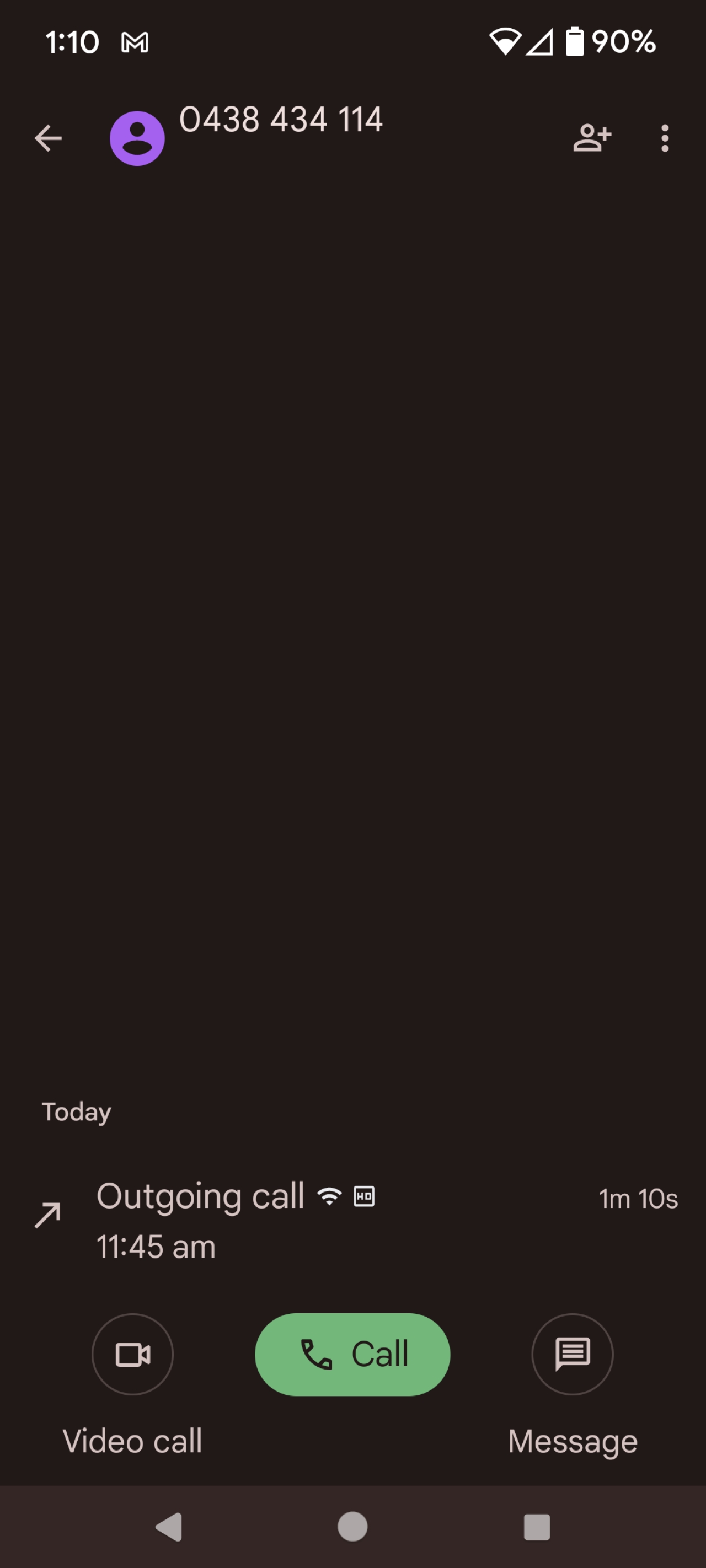This detailed screenshot, taken from an Android device, showcases the user's call history and interface options. The screenshot reveals that the user first made a call to the number 0438 434 114 at approximately 1:10 AM. A subsequent outgoing call was placed at 11:45 AM, lasting around 1 minute and 10 seconds. The call button is highlighted in green for emphasis, accompanied by additional options for video calling and messaging, both presented in white text.

Additionally, there are three primary navigation buttons at the bottom: a white triangle (indicating the back function), a home circle (currently pressed), and a white square for accessing further options. 

At the top of the screenshot, indicators show that the phone's battery is at 90% and the device is connected to the home WiFi network. The interface background is presented in a dark brown hue, while the bottom navigation bar features a lighter brown color. 

Finally, the call button's green background serves to highlight its importance to the user on this touchscreen interface, contrasting sharply with the black and grey text to draw attention.